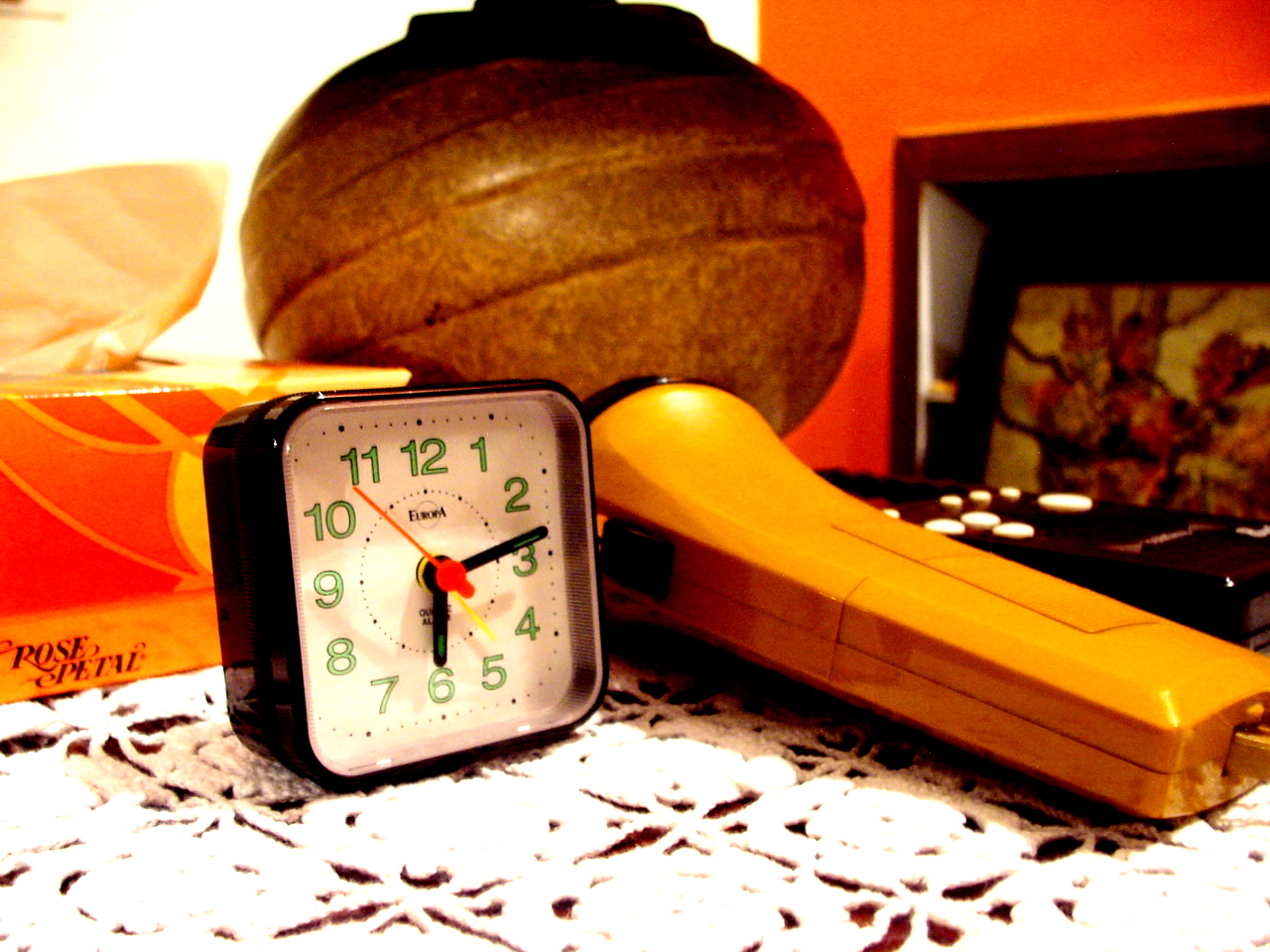This image depicts a detailed and nostalgic scene centered around an old-fashioned analog alarm clock. The clock, square in shape with a black plastic body and a white face, displays the time as 6:13. It features glowing green numbers, black hour and minute hands, and a distinct red second hand. Positioned on a table covered with a white lacy tablecloth, the clock is surrounded by various retro items adding to the ambiance. To the clock's right lies an orange plastic device, potentially a flashlight, characterized by a wider top and a smaller, rectangular body. A brown vase, which doubles as the base of a lamp, stands behind these objects, contributing an elegant touch with its spherical shape and brown tint.

The table is further adorned by a box of Rose Petal tissues, noticeable with its orange-yellow hue and white tissues protruding at the top. The tissues, capturing the vintage palette of the scene, appear slightly yellow due to the overall orange tint of the photograph. The background reveals an orange wall to the right, with a blurry image or artwork, while the left side features a dark, possibly brown, area that could be a fireplace. The image, enveloped in a warm, orange tint, lends a homely, retro feel to the entire setup, making it a snapshot of vintage charm.